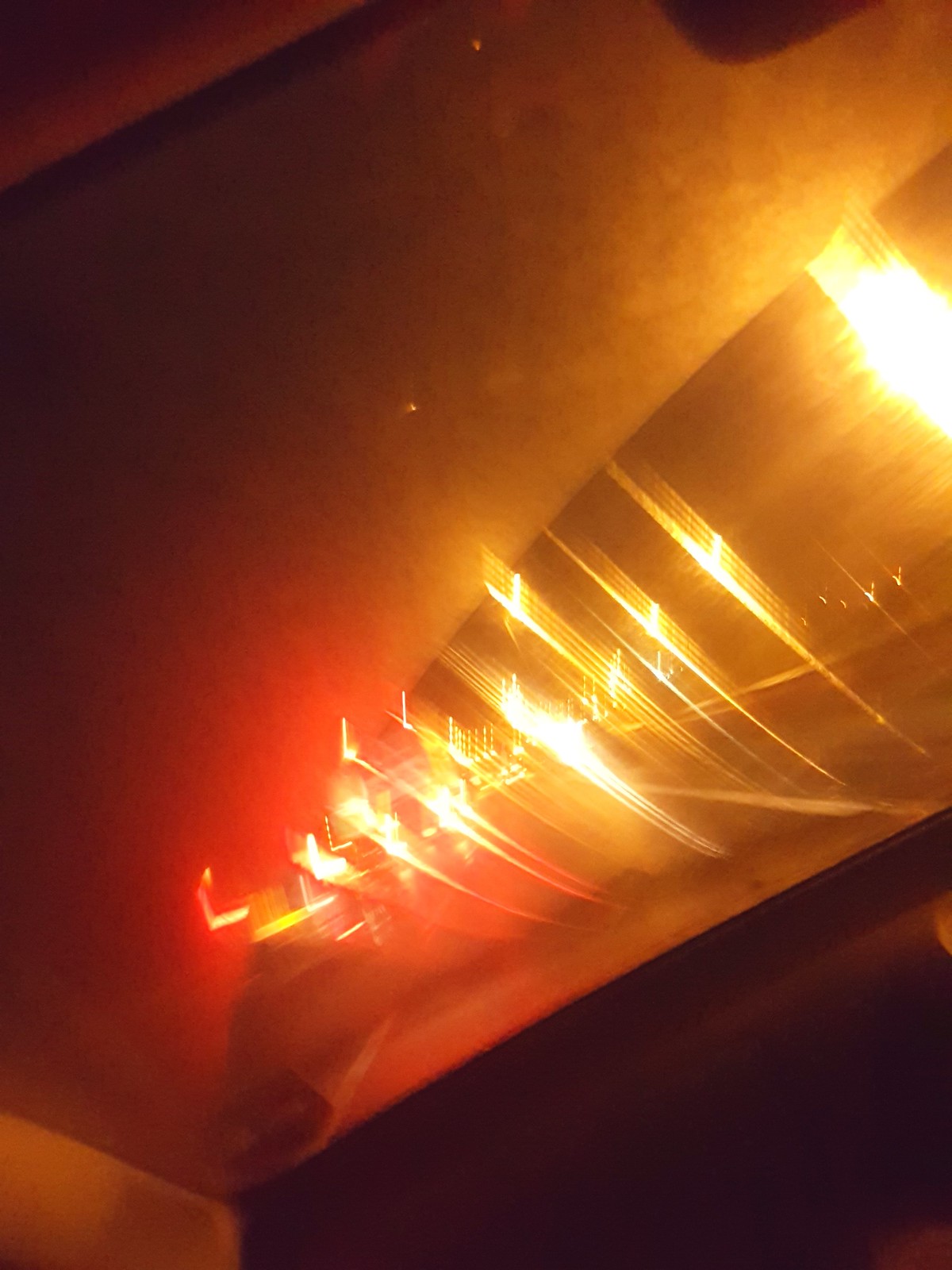This photograph captures the misty, reflective view from inside a car, possibly from the front passenger seat or the backseat. The main focus is the car window, which appears partially fogged up due to external humidity. Through the clear portions of the window, one can glimpse blurred headlights and streetlights, suggesting the vehicle is navigating through traffic. Subtle reflections on the window, likely from the dashboard, intensify the sense of closeness to the dash, though it’s not entirely clear which seat you’re in. The ambient light outside casts a warm, orange-yellow glow, illuminating parts of the road and its white lines. The overall scene exudes a sense of moving through a luminescent urban landscape.